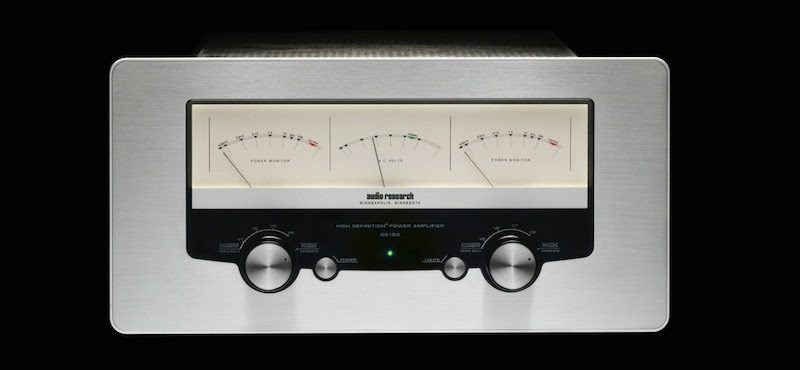The image shows a detailed high-definition power amplifier by Audio Research placed on a large horizontal black rectangle. The amplifier itself is a shiny silver metal rectangle and is adorned with several intricate features on its face. 

Dominating the front of the amplifier, there are three gauge-like dials reminiscent of fuel gauges in a vehicle, used to measure sound levels. These gauges feature black lines that move from left to right to indicate various readings. Surrounding these gauges is a combination of black and a dull white background, adding to the device's aesthetic appeal.

Beneath the gauges, a prominent silver strip runs horizontally across the front. This strip bears black lettering at its center, including the words "high-definition power amplifier," along with the brand name "Audio Research" and location-related text. The front panel of the amplifier also includes four buttons – two large and two small – all black with silver tops and surrounded by white text on a black background. 

In the very center of the amplifier, amid the buttons, a green light signifies the device's operational status. This nuanced design and array of controls underline the device's sophisticated functionality and high-end audio processing capabilities. The background of the image remains completely black, helping highlight the amplifier's sleek, modern design.